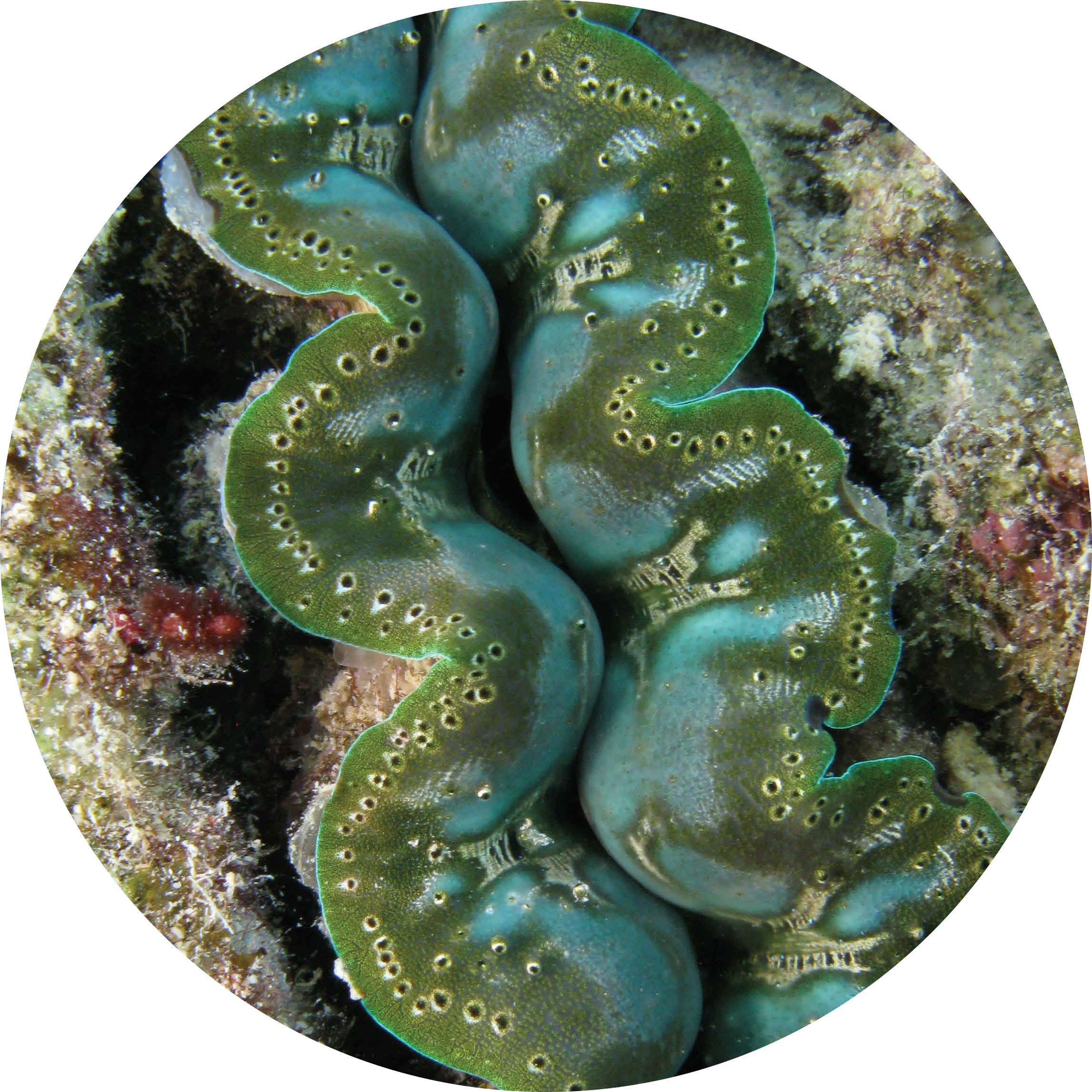This circular image, resembling something you might see in a Petri dish, features two prominent, worm-like creatures that extend from the top to the bottom of the frame. These creatures are green and blue, with a series of small black holes dotting their surfaces, giving them a caterpillar or slug-like appearance. They are curved and positioned closely together, almost touching, creating an 'S' shape. Surrounding these creatures on the left and right sides is a porous, quartz-like substance with speckles of white, red, and some green. The background behind these worm-like figures and the porous material is solid black, providing a stark contrast to the more detailed elements in the image. Although the exact nature of the scene is unclear, it suggests an underwater or microscopic view, possibly showing organisms pressed against a glass surface.